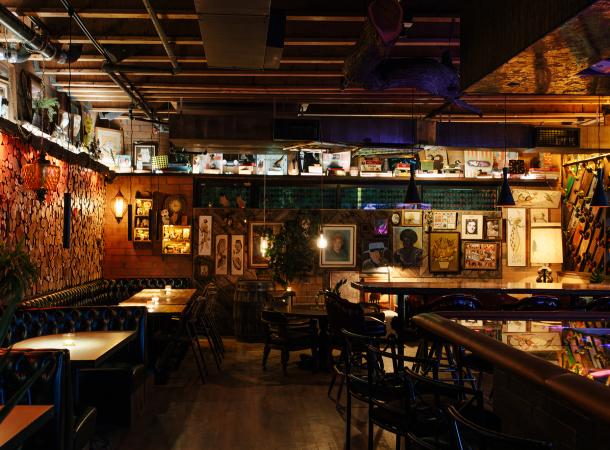The image depicts an indoor scene of a moody, artsy bar or restaurant with a distinct warehouse vibe. The ambiance is dark and characterized by earth tones, giving it a sepia, almost nostalgic feel. On the left side of the image, there are several leather-padded booths with tables in front of them. The right side features a bar area with stools, although the bar itself is somewhat out of the main focus. The ceiling is exposed, revealing pipes, AC units, and wooden slats, contributing to the industrial aesthetic. Various pictures and paintings line the back wall, extending from left to right, adding bursts of color to the otherwise subdued palette. Additionally, there's a shelf running across the top of the room, showcasing an assortment of memorabilia. The room appears empty, suggesting the place might be closed at the time the photo was taken.